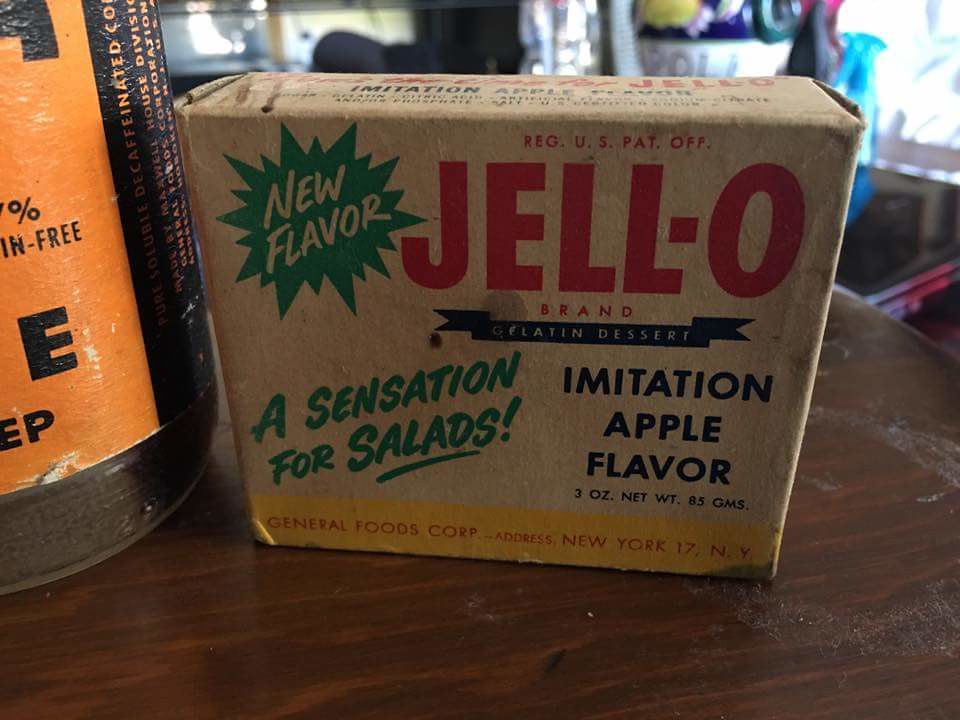This indoor color photograph captures a close-up of a very old-fashioned Jell-O package, positioned prominently on a worn, dark brown wooden tabletop with white powdery stains. The rectangular box, made from brown cardboard, features a nostalgic design with various colored fonts and elements that give it a vintage appearance. 

At the top of the package, a green starburst shape announces "New Flavor." Below this, in large red letters, it says "Jell-O," with "Brand" written directly underneath in a smaller font, followed by "Gelatin Dessert" on a green banner. The package prominently highlights its "Imitation Apple Flavor" in a dark blue font and specifies "3 oz. net weight." In a playful, slightly tilted green script, it also reads, "A Sensation for Salads!" In smaller text along a yellow stripe at the bottom, the box states its manufacturer: "General Foods Corp., New York 17, N.Y."

The setting includes an additional object—a cylindrical coffee can with an orange label—positioned to the left of the Jell-O package. The background reveals a cluttered sink area with indistinguishable details, while light filters in from the right. The entire scene is dimly lit, emphasizing the well-preserved but clearly aged Jell-O box as the central focus of the image.